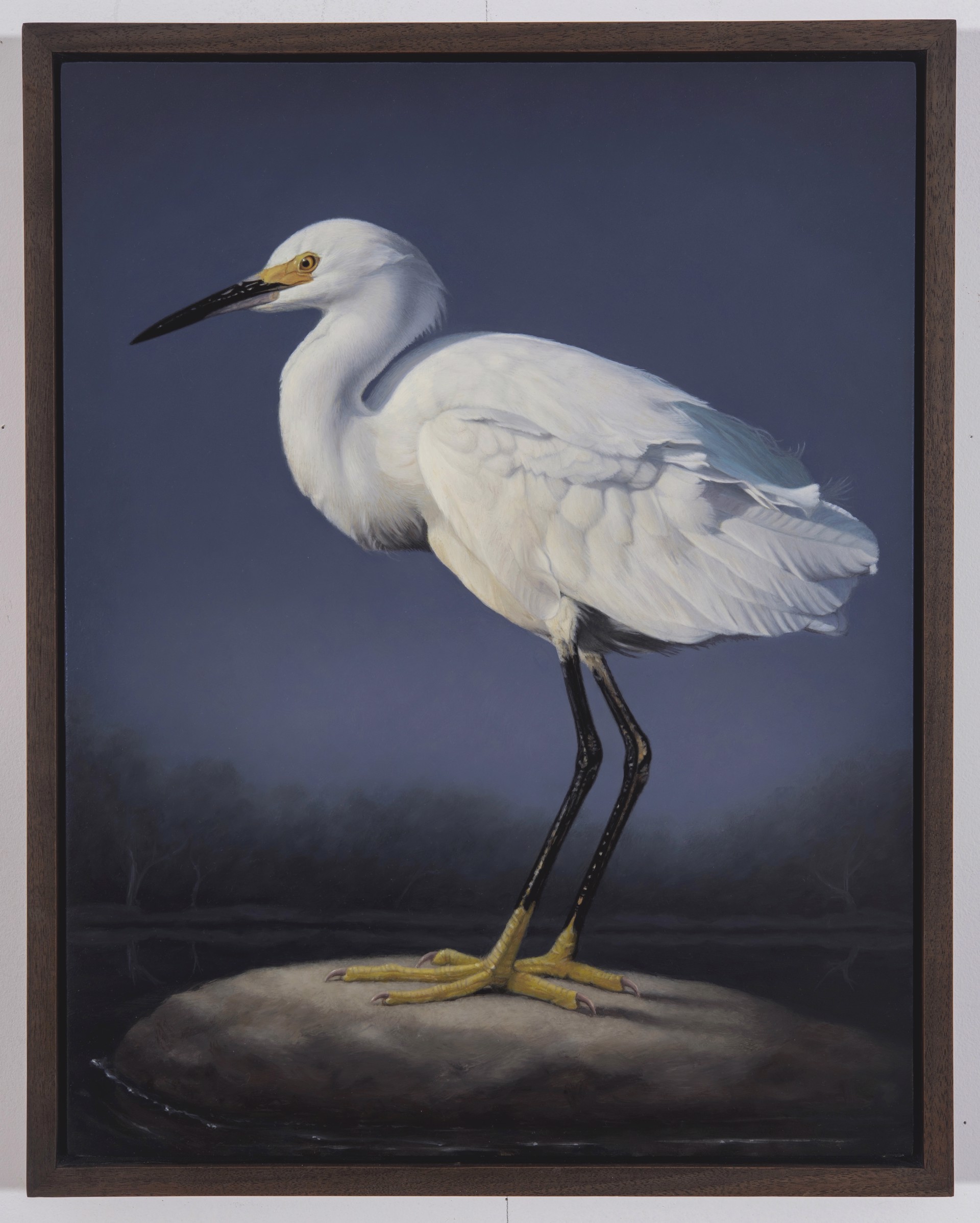The image showcases a meticulously detailed, photorealistic painting of a bird, likely a swan, standing gracefully on a gray rock amidst a body of water, such as a pond or river. The bird, predominantly white with darkened feathers under its neck, features long, slender black legs and yellow feet that touch the rock. Its long black beak, about the size of its head, is accentuated by yellow markings around its eyes, giving it a striking appearance. The eyes themselves are yellow with black pupils. The serene background portrays a dark, overcast sky, possibly indicating twilight, with a faint hint of dark blue near the horizon, suggesting the sun is either setting or rising. A row of windswept trees stretches across the horizon, adding to the tranquil yet slightly somber mood of the scene. The entire composition is framed by a brown border, and there is no text present in the artwork.